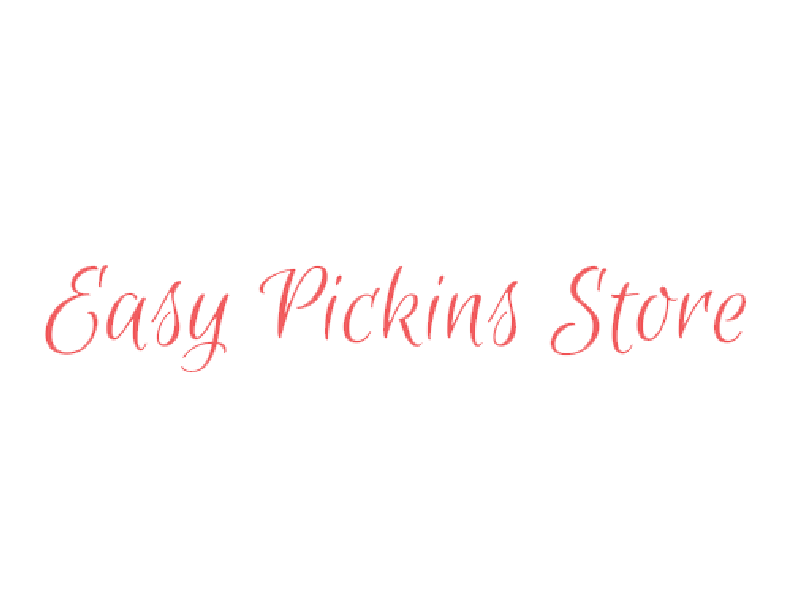This image features a logo with no border, set against a pure white background. The logo consists of three distinct words written horizontally from left to right: "Easy," "Pickins," and "Store." Each word is rendered in a thin, fine cursive script with a noticeable low-resolution quality, resulting in jagged, blocky edges. The text color is a vivid pinkish-red. Each line of text starts with an uppercase letter followed by lowercase letters: 'E' in "Easy," 'P' in "Pickins," and 'S' in "Store." Additionally, the 'I' in "Pickins" has red dots over it. The letters are not connected to each other.